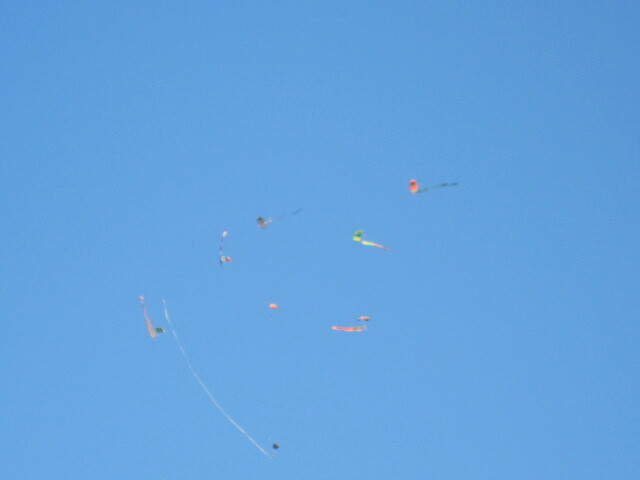In this vibrant and clear image, a dazzling array of kites dances in a cloudless, bright light blue sky. The photograph captures the scene from a considerable distance, making the kites appear as colorful, indistinct shapes against the consistent blue backdrop. Among the assortment, vivid hues of red, yellow, and orange stand out, alongside a spectrum of other colors including green and pink. Notably, one kite features an extremely long, curving white ribbon tail, while others boast similarly lengthy tails streaming behind them. Though the kites are too far away to discern precise details, their lively presence and varied forms create a captivating display.